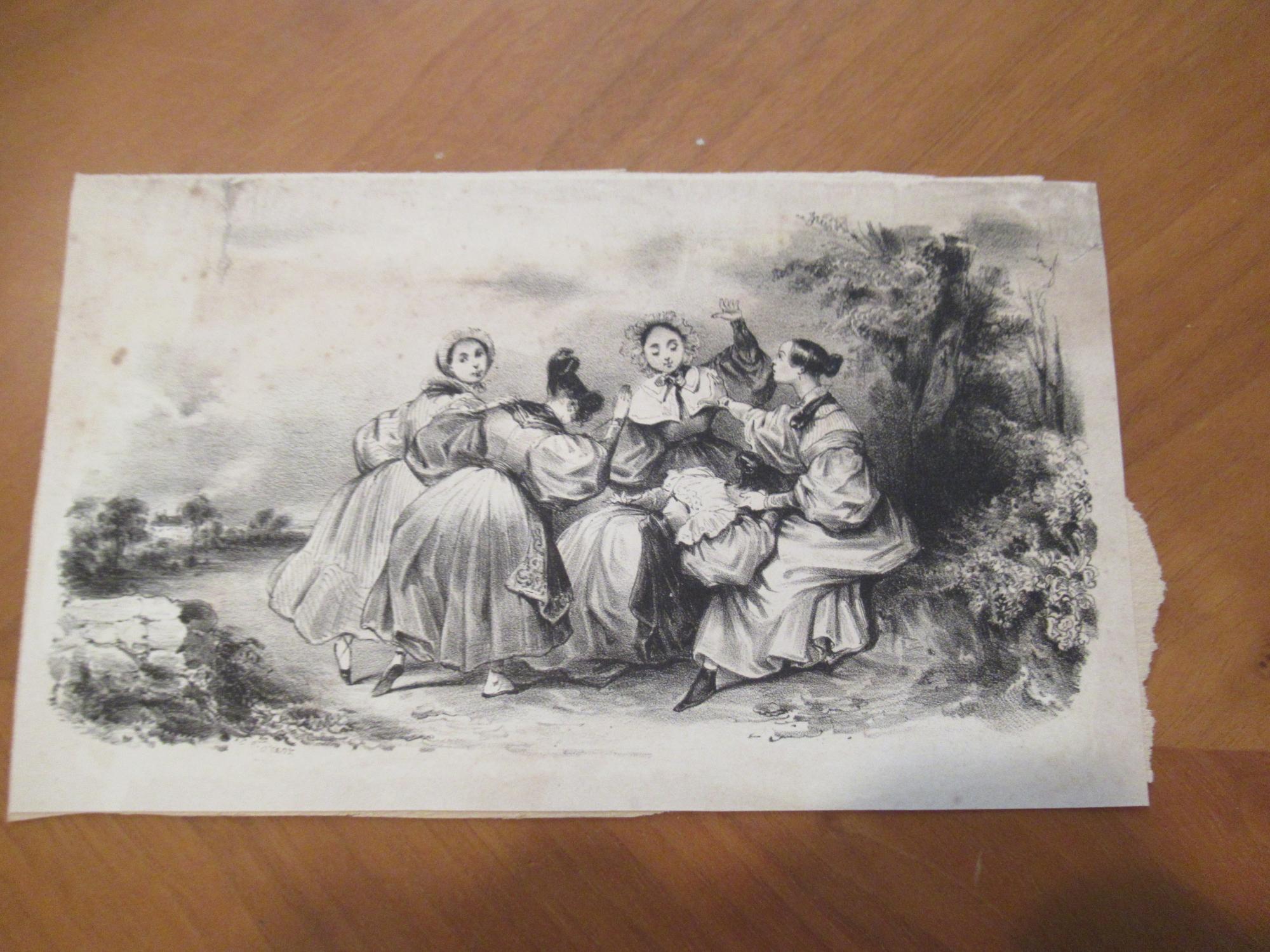This black-and-white drawing, possibly created with charcoal on white paper, portrays four women in what appears to be a celebratory or dancing scene set in an outdoor area adorned with foliage, including trees and small shrubs. The image, which rests on a brown wooden surface and has some tearing on its bottom right edge, is a testament to its age, suggesting it might be from the 1700s or 1800s. The woman on the far left, who wears a bonnet and pointy or ballerina-like shoes, is turned to look over her shoulder at the viewer. The second woman, facing away from us with her hair in a bun, also seems to be dancing in a long white dress. The third woman, positioned centrally, is dressed similarly and has her right hand in the air, appearing to be mid-dance. The fourth woman on the far right, with her hair pulled back, reaches out to her companion, looking up with an expression of supplication. Despite the lack of much background detail, the shrubs and trees add depth to the composition, enhancing this evocative scene of historical elegance and motion.